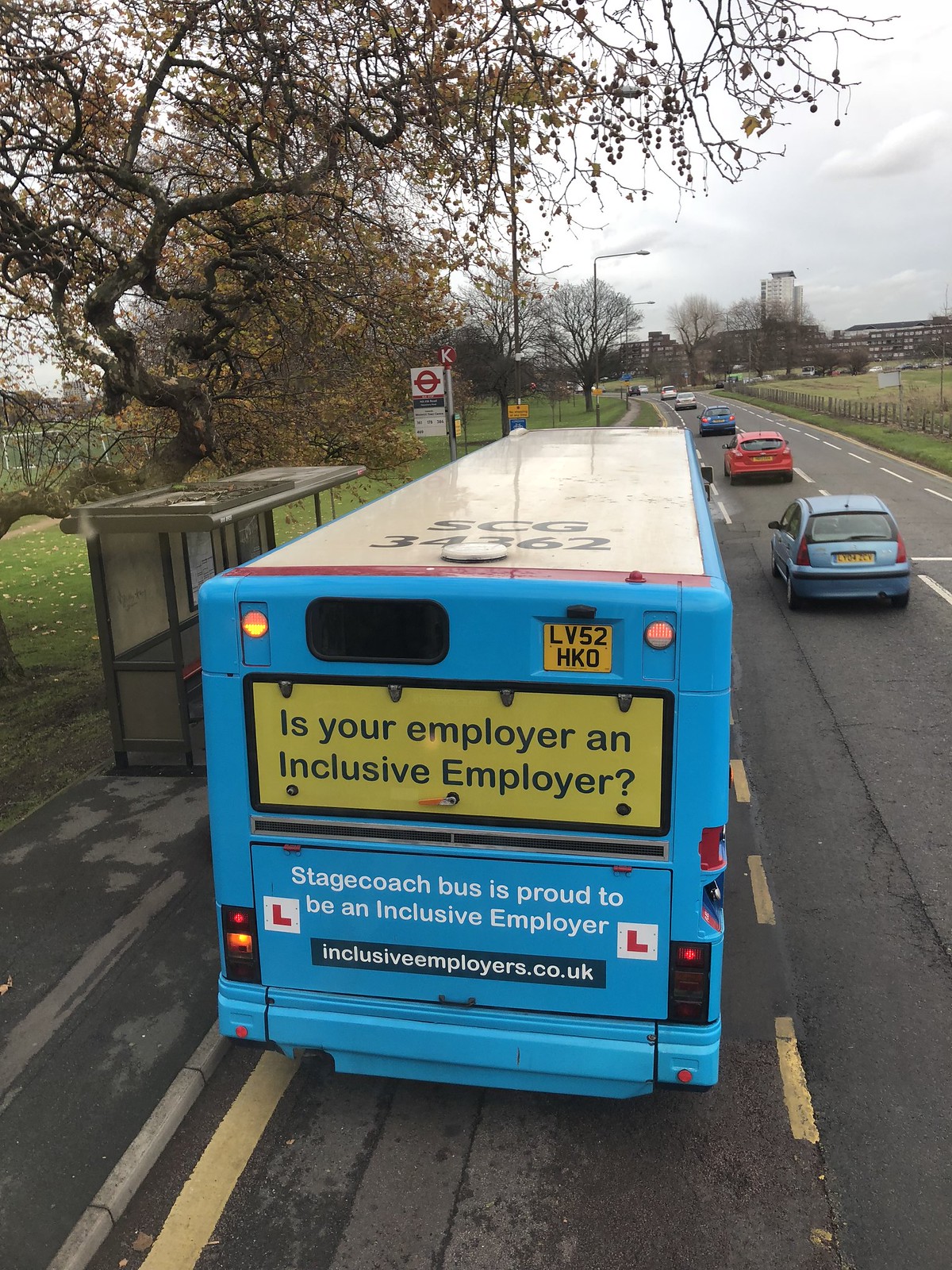This is a detailed color photograph depicting a roadway scene on a dark, cloudy day. The weather suggests it might be late fall. The main focus of the image is a blue bus, prominently displayed from the rear view. The bus is stationed at a small bus stop, seemingly in the process of picking up or dropping off passengers. The bus has a distinctive white roof with black text and bears an orange license plate with black text in the upper right-hand corner. A prominent yellow banner dominates the back with bold black lettering asking, "Is your employer an inclusive employer?" Directly beneath, white text on a blue background declares, "Stagecoach Bus is proud to be an inclusive employer." Below that is a black banner with white text that reads, "inclusiveemployers.co.uk," flanked by red 'L' symbols in white squares on either side.

To the left of the bus, a bus stop shelter and a tree with greenish-brown leaves can be seen. The right side of the image shows a road with multiple cars—blue, red, and silver—driving in the distance. Yellow and white lines mark the asphalt road, contributing to the scene's overall structure and directing the flow of traffic.